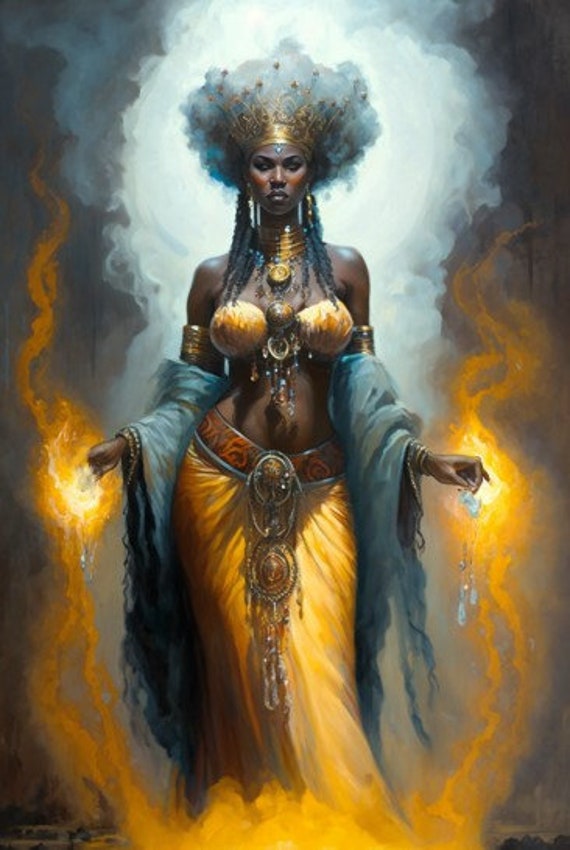This is a detailed artistic painting depicting a powerful African-American woman, possibly an embodiment of an Egyptian or Western African goddess. She is adorned with a magnificent golden headdress, intricately styled with gray and black feathers or flowers, evoking the aura of a priestess or a mystical figure. Her long black dreadlocks cascade from the crown, framing her full face, accentuated by elaborate makeup and a touch of red rouge. A jewel graces her forehead, and bangles and bracelets adorn her arms, enhancing her regal presence.

She wears a striking orange-yellow bikini top and matching skirt that shimmer like fire, symbolizing her potent power. Around her waist, a large ornate belt with intricate symbols and giant colored stones hangs down, adding to her imposing demeanor. A light bluish shawl drapes over her arms and wraps behind her, contrasting with her vibrant outfit and drawing attention. 

In her hands, she clasps feathers, and flames rise at her feet and ascend around her, emphasizing her connection to fiery, mystical powers. A long necklace with various gold, white, and silver ornaments trails down her chest, extending past her knees, further highlighting her divine and authoritative presence.